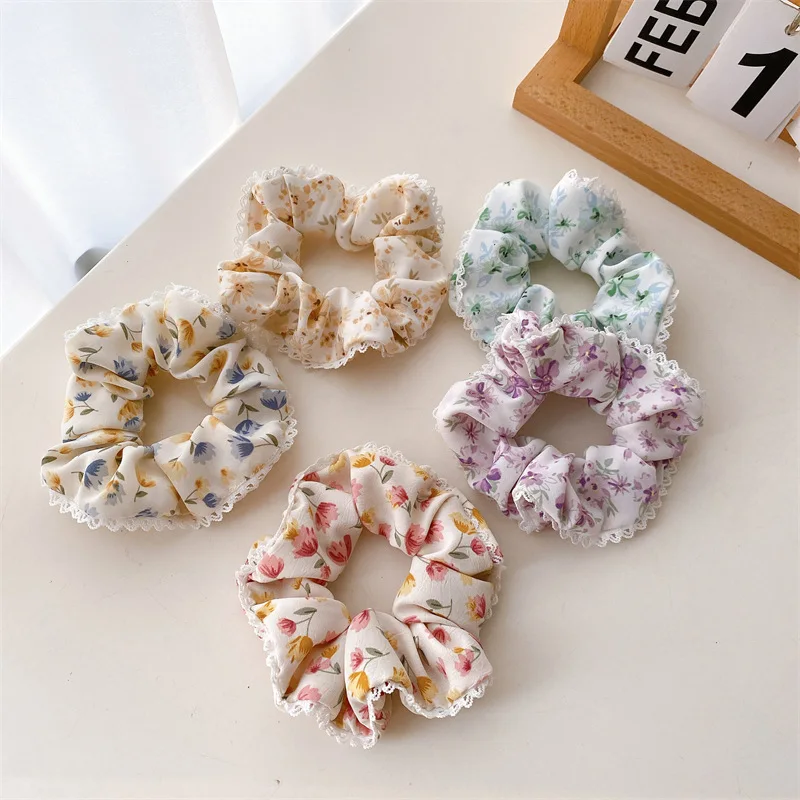This is a high-angle promotional photograph featuring five different floral-patterned hair scrunchies, each detailed with white lace around the edges. From left to right, the scrunchies display vibrant colors and patterns: the top left exhibits blue flowers, the top center is adorned with mustard-colored floral designs, the top right shows green flowers, the right one has purple flowers, and the bottom one combines pink and yellow flowers. These scrunchies, all seemingly made of fabric with elastic bands, are arranged atop a white tabletop surface. A partially visible calendar at the top shows the date February 1st, made of light brown wood with black paint, indicating a customizable date display. The background features what appears to be a white curtain, suggesting a cozy, indoor setting.